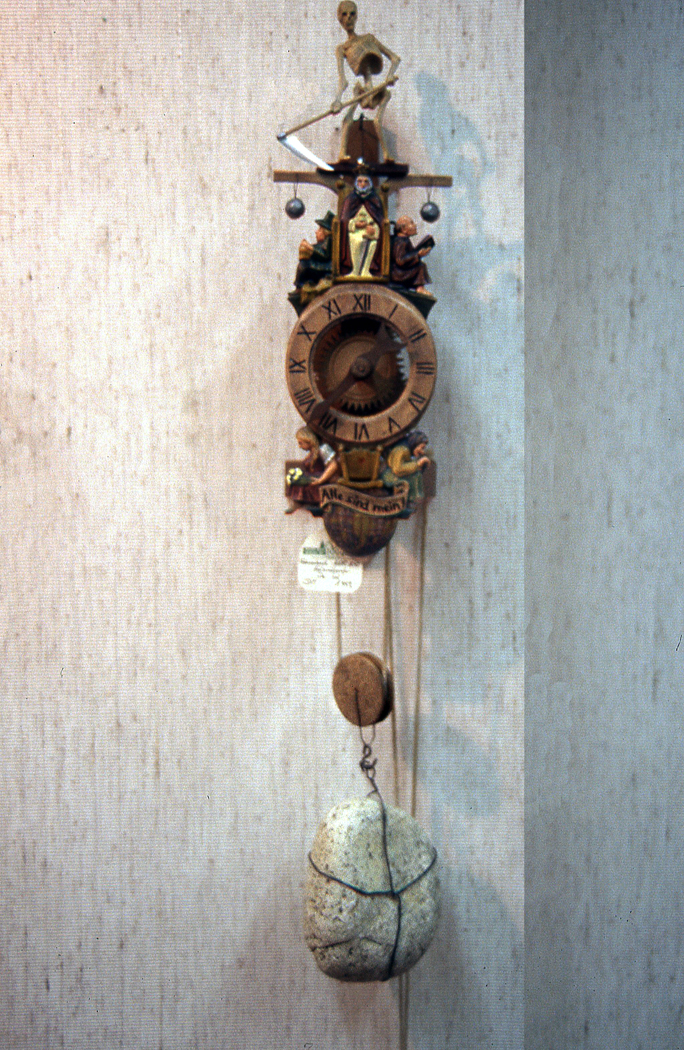The image showcases a very unique and artsy wooden clock mounted on a gray wall. The clock features an ornate design extending from the top of the wall down to the middle. At the very top of the clock, a skeleton, resembling the Grim Reaper, faces toward the camera while holding a scythe. The handle of the scythe stretches to the left, and the blade curves back to the right diagonally downward. Just below the skeleton, there is a cross with two black balls hanging from its horizontal arms. 

Continuing down the clock, below the cross, is a man in a blue shirt and white pants who is facing toward the viewer. On either side of him, there are two seated figures—one on the left, dressed in black clothes and a black hat, facing left; and one on the right, facing in the opposite direction. Below this central figure is the clock face itself, which has a wood grain finish and features Roman numerals around its edge, with a dark brown center and matching numbers. 

Below the clock face, there are two women positioned on the left and right sides, each gazing in opposite directions: the woman on the left faces left, and the one on the right faces right. Further down, a small curved hump supports a banner, and two strings hang down from either side of this feature. These strings are connected to a wooden pulley that holds a large gray-white rock with strings draping over its front and sides. The overall design of the clock and its intricate details, including human figures, religious elements, and mechanical components, contribute to its highly artistic and intriguing appearance.